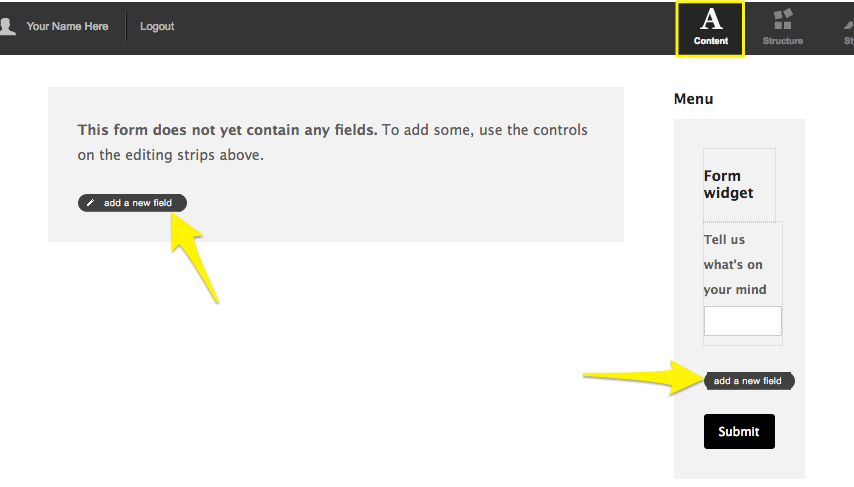Screenshot of a productivity website interface with a black header and features for form creation:

In the black header, the top left corner displays two tabs titled "Your Name Here" and "Logout." The right side of the header features three icons: an 'A' (representing content), a structure icon, and a content/tag icon, which is highlighted with a yellow box. The main content area below the header is primarily white.

There are two primary sections in the interface:

1. **Main Form Area**: 
    - Occupies the majority of the space.
    - Contains the message: "This form does not yet contain any fields. To add some, use the controls on the editing strip above."
    - A black "Add a New Field" button is centrally located with a yellow arrow pointing towards it from below.

2. **Sidebar Menu**:
    - Positioned on the far right.
    - Titled "Menu" at the top.
    - Contains a titled section "Form Widget" with the prompt "Tell us what's on your mind."
    - Beneath the prompt is a white input bar for user input.
    - Below the input bar are two buttons:
        - A black "Add a New Field" button with a yellow arrow pointing towards it from the left.
        - A black "Submit" button.

The remaining portions of the webpage are blank with a white background.